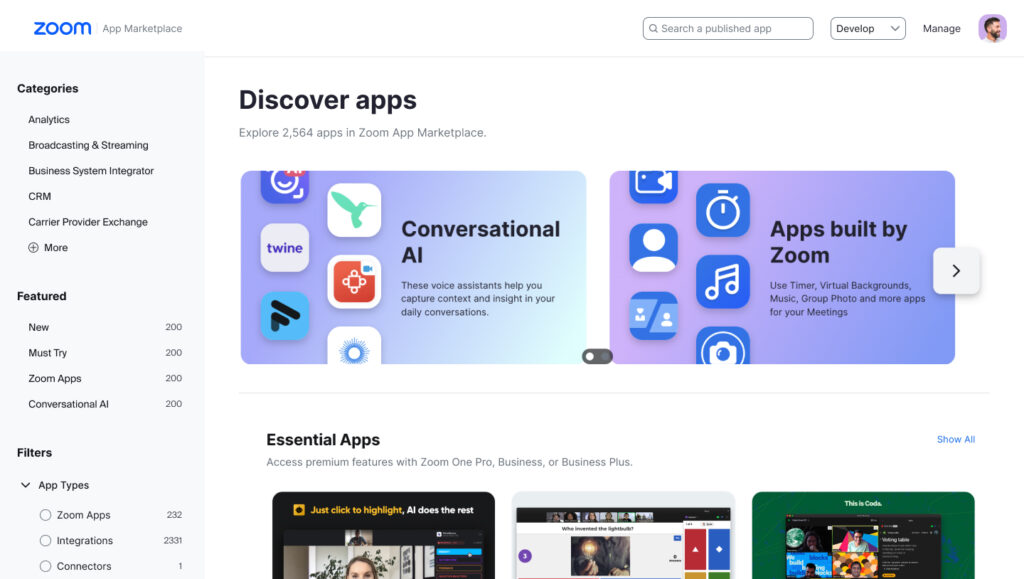The landing page for Zoom's App Marketplace features a well-organized layout. In the upper left corner, the familiar Zoom logo appears in blue, followed by the text "App Marketplace" in small gray letters to the right. At the top center of the page, a search bar prompts users with the placeholder text "Search a published app." Next to the search function, a navy blue button labeled "Develop" is accompanied by a dropdown menu. Further to the right, the "Manage" option is displayed, followed by the user's profile picture, which shows a profile view of a man with dark hair, a beard, and a mustache.

A very pale gray line runs horizontally beneath this top section, providing separation from the main content. On the left margin, a wide ribbon in a light blue or light gray color showcases primary navigation options. At the top of this ribbon, the bold black text "Categories" is prominently displayed. Indented underneath are options such as "Analytics," "Broadcasting and Streaming," "Business Systems Integrator," "Carrier Provider Exchange," and a "More" option with a plus sign.

Below the categories, the bold black text "Featured" introduces sections like "New," "Must Try Zoom Apps," and "Conversational." A final category, "Filters," also includes a dropdown in bold black text labeled "App Types," with indented options like "Zoom Apps," "Integrations," and "Connectors."

In the main section of the image, bold black text at the top reads "Discover Apps," followed by gray text that states "Explore 2,564 apps in Zoom App Marketplace." The page features various colorful boxes that provide additional information about the different apps available.